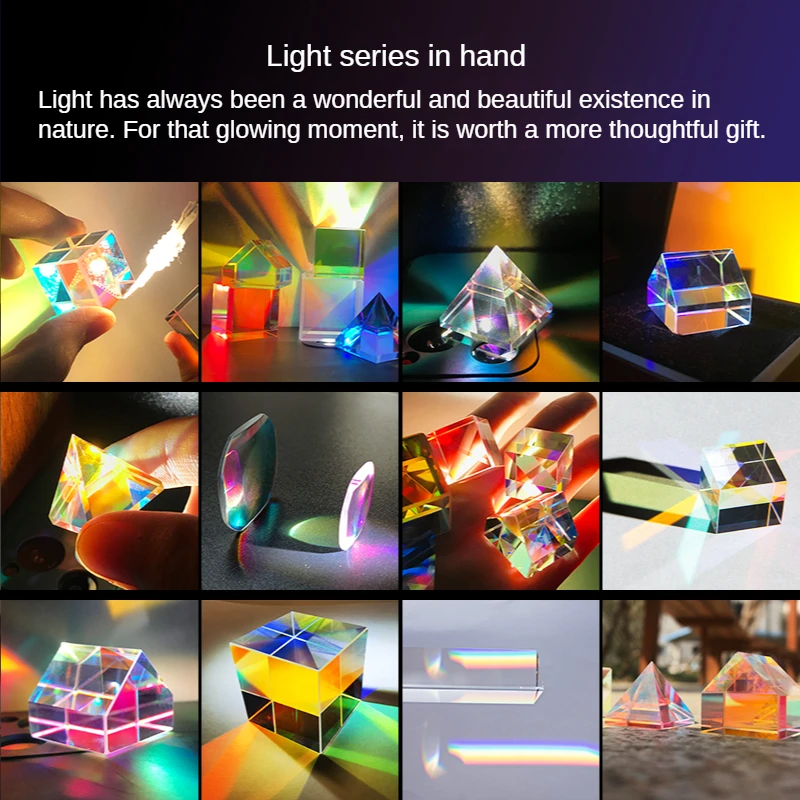This detailed image features a dark background with white writing that reads, "Light Series in Hand. Light has always been a wonderful and beautiful existence in nature. For that glowing moment, it is worth a more thoughtful gift." It appears to be either an infographic or a PowerPoint presentation showcasing the fascinating effects of light when interacting with various prisms and light-up cubes. The layout consists of twelve boxes arranged in three rows of four columns.

Each box contains a vividly detailed image of prisms and cubes in different shapes and sizes, demonstrating how they manipulate light to produce beautiful multicolored effects. Some prisms are shaped like perfect cubes, while others resemble pyramids, spheres, or even tiny houses. The images include scenarios such as a light-up cube being delicately pinched by fingers, cubes sitting on desks, prisms held over iPhone flashlights, and clusters of small, glowing prisms emitting a spectrum of colors like white, green, blue, orange, red, and purple.

Throughout the infographic, these prisms and cubes are depicted in a variety of arrangements: some are showcased individually, others in groups, and some are held by hands, which highlight their small size. The images aim to capture the enchanting essence of light as it interacts with these geometric shapes, creating a captivating and thoughtful visual experience.